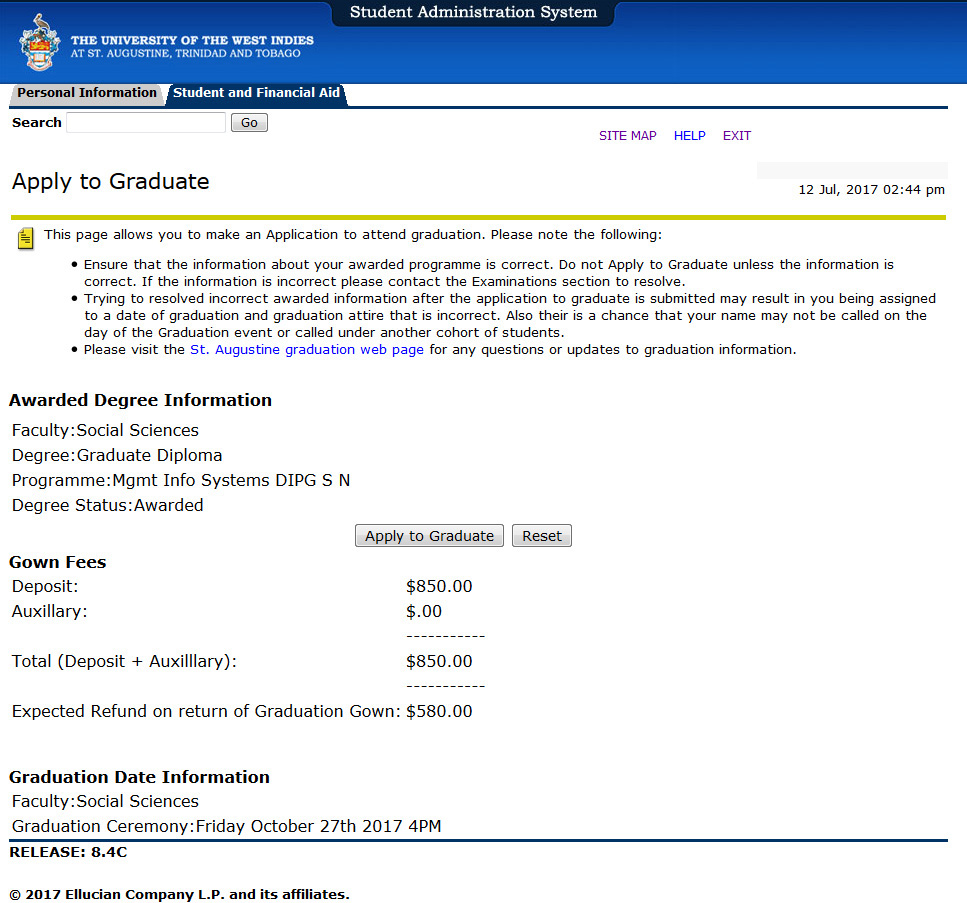The image depicts an official letter from the University of the West Indies, St. Augustine campus in Trinidad and Tobago. The letter features a blue border at the top, prominently displaying the university's name on the upper left. Below this, the text highlights two tabs: 'Personal Information' and 'Student and Financial Aid'. 

Next, the document provides instructions headed "Apply to Graduate". A brief explanatory note states: "This page allows you to make an application to attend graduation. Please note the following," followed by three bullet points. The first bullet point urges students to "ensure the information about your awarded program is correct." The second explains that attempting to resolve incorrect awarded information after submission "may result in you being assigned an incorrect date of graduation and graduation attire." The third bullet advises students to visit the St. Augustine graduation webpage for queries and updates.

Further down, there is a section titled "Awarded Degree Information." Here, the details read: "Faculty: Social Sciences, Degree: Graduate Diploma Program, Major: Management Information Systems, Degree Status: Awarded." Below this section, an "Apply to Graduate" button is displayed, along with a "Reset" button.

Additionally, under "Gown Fees," the letter specifies that a deposit of $850 is required, with a total of $580 expected to be returned upon the return of the gown.

Towards the lower portion, the document provides "Graduation Date Information," stating that the Faculty of Social Sciences' graduation ceremony is scheduled for Friday, October 27, 2017, at 4 p.m.